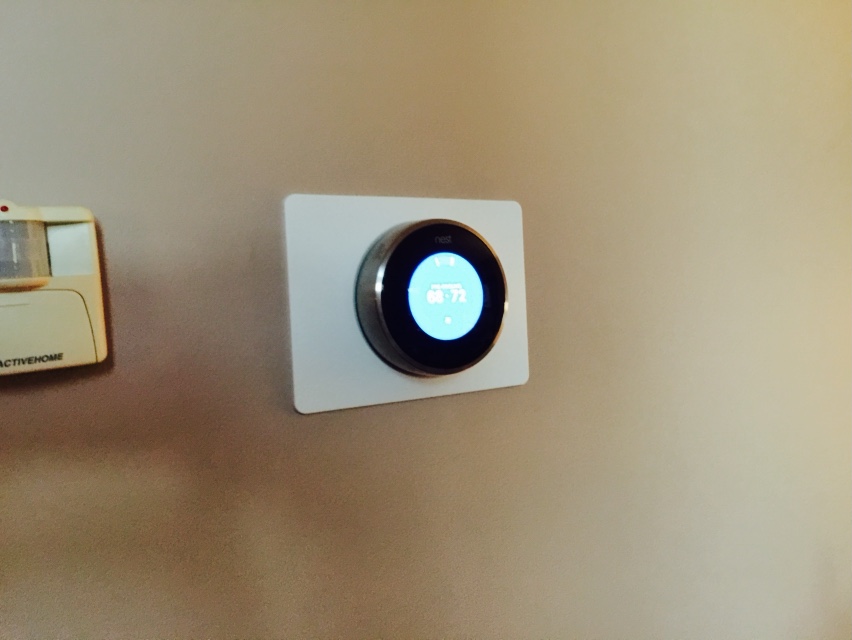The image features a prominently centered white rectangular piece, either plastic or metal, with smoothly rounded edges against a very blurry background. In the middle of the rectangle, there's an elevated black circular disc that encases a light blue interface, likely glass, emitting faint illumination. The light blue section displays white numbers, though they are somewhat indistinct. Adjacent to this central figure, towards the left edge of the image, there's an off-white or yellowish object resembling a thermostat box. The bottom of this smaller box bears the marking "Active Home."